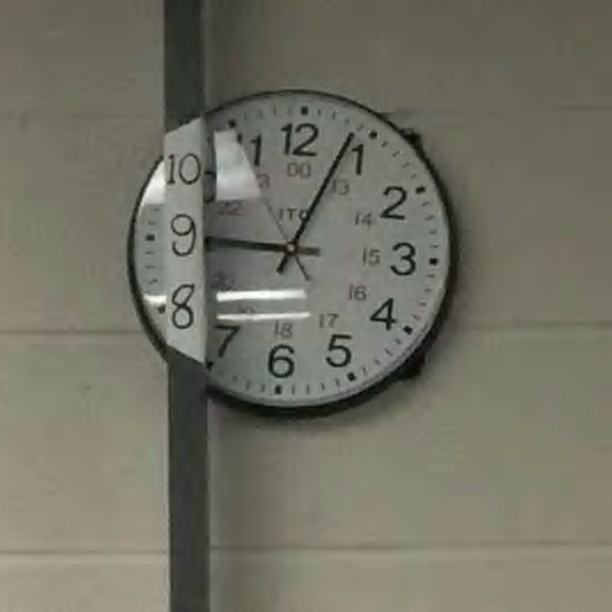The image showcases a white concrete block wall, uniformly painted in white. Mounted on this wall is a standard, round clock with a black casing and white face. The clock features black numerals and hands, embodying a classic design. Intriguingly, a vertical metal bar extends from the floor to the ceiling, intersecting the clock and obscuring the numbers 8, 9, and 10.

To address this obstruction, someone ingeniously painted over the metal bar covering the clock. They recreated the clock’s white background on the metal surface and carefully added the numbers 10, 9, and 8 in black, aligned vertically. This thoughtful addition enables viewers to discern the hidden portions of the clock’s face, thereby restoring its function and ensuring that the timepiece remains legible despite the physical barrier.